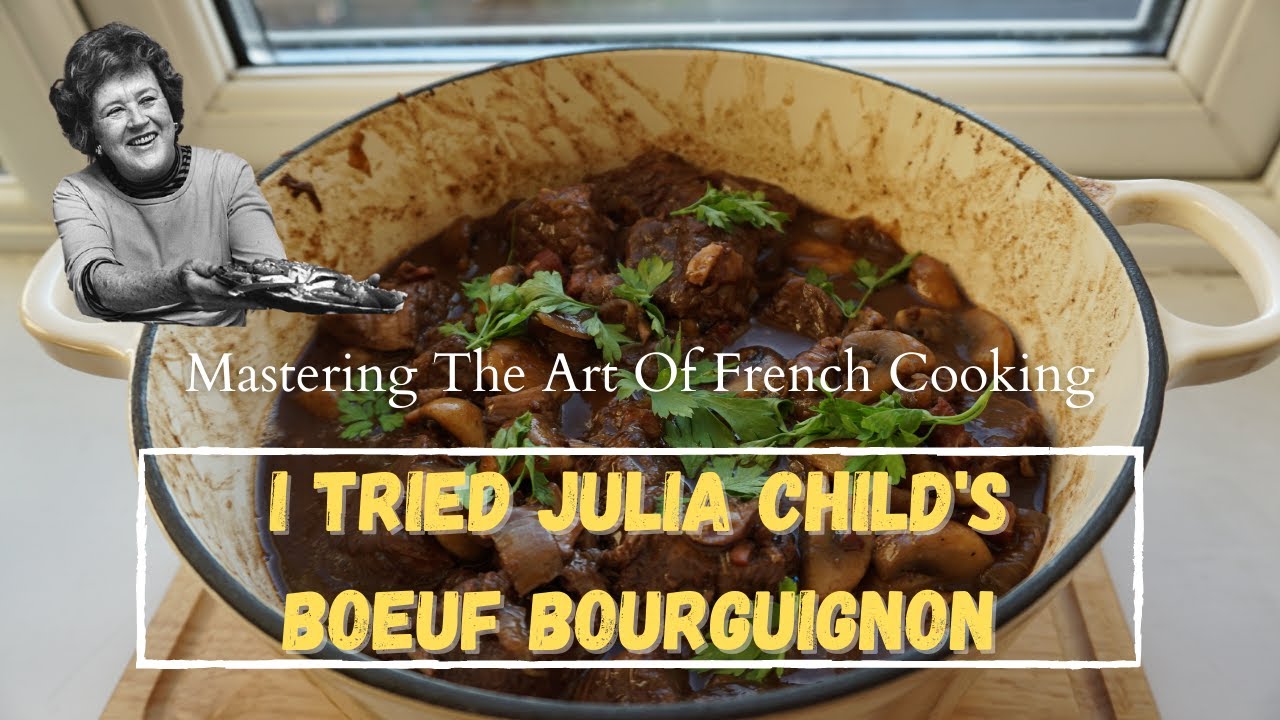The overhead image appears to be a thumbnail for a YouTube video or a banner for a food blog, showcasing a culinary dish prepared in a circular white pot with a black ring around the top edge. The pot contains dark brown beef in a rich, dark brown sauce, with green herbs such as parsley or cilantro sprinkled on top. The sauce has splashed onto the inner sides, leaving noticeable stains. The pot features rounded handles on both sides; the handle on the left side displays a black-and-white photo of Julia Child from the waist up, dressed in a gray shirt with outstretched hands holding a silver platter. Superimposed text on the image reads, "Mastering the Art of French Cooking." Below this, a white text box with yellow text states, "I tried Julia Child's Boeuf Bourguignon." The composition, with its detailed focus on the dish and the clear textual elements, is ideal for a YouTube thumbnail or a food blog header.